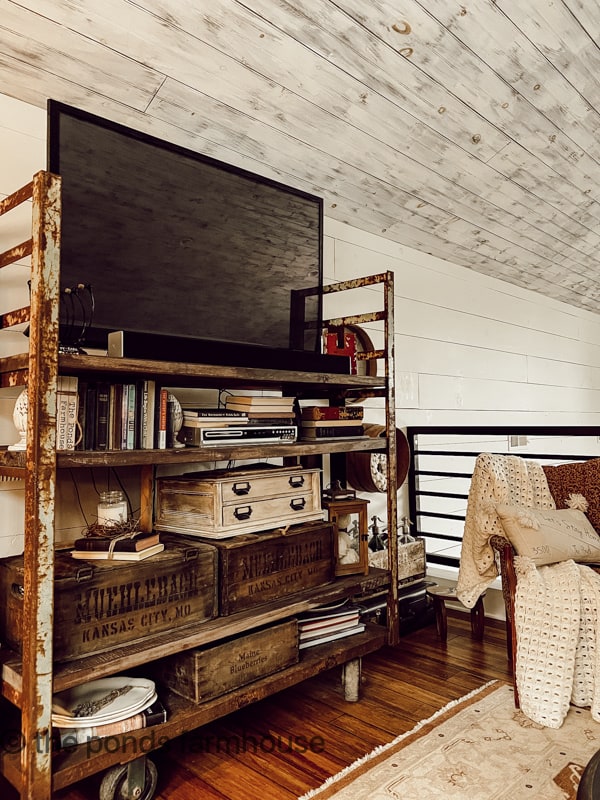The image depicts an earthy-toned interior with a light oak ceiling creating a cozy ambiance. In the lower right corner, a third of a chair can be seen, adorned with a cream-colored afghan and pillow. This chair sits on a cream area rug with a gold border, which lies over a wooden floor. A rustic, distressed-looking metal cart on wheels has been repurposed as a shelf. The shelf hosts various bins and boxes, a row of books, and a large TV on top, estimated to be around six feet wide. Below the TV are more books, antique-style boxes, and dishes, all contributing to a western 1800s aesthetic. In the background, a balcony is visible, suggesting this cozy space is located on the second floor.